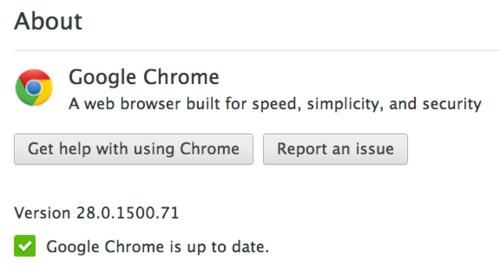In this image, set against a solid white background, the upper left corner features dark gray bold text stating "Google Chrome." Directly beneath the text, a narrow gray horizontal line runs across the width of the image. On the left side below this line is the Google Chrome icon, which consists of a round circle segmented into the colors yellow, red, blue, and green. Accompanying the icon, there is a descriptive phrase: "Google Chrome, a web browser built for speed, simplicity and security."

Below the icon are two gray action buttons with dark gray text and a light gray outline. The button on the left is labeled "Get help with using Chrome," while the button on the right reads "Report an issue." Below these buttons, in smaller gray text, the version number "28.0.1500.71" is noted, followed by the message "Google Chrome is up to date."